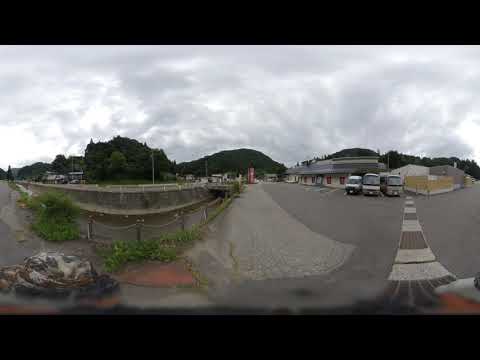The image captures a gray, overcast sky hanging over a panoramic view of a parking lot and a roadway. The scene is framed by thick black borders at the top and bottom. The road, made of gray pavement, divides the image horizontally with a distinct stripe running down the center. To the left, a rock wall curves U-shaped with bushes and some rocks in front of it. On the right side, parked vehicles including two trucks and a van face a tan, one-story building with maroon window frames. The trucks are white with large windshields, and the low hills covered in green trees and bushes are prominent in the background. Over half of the image is dominated by a cloudy, gray sky, giving the sense of impending rain.